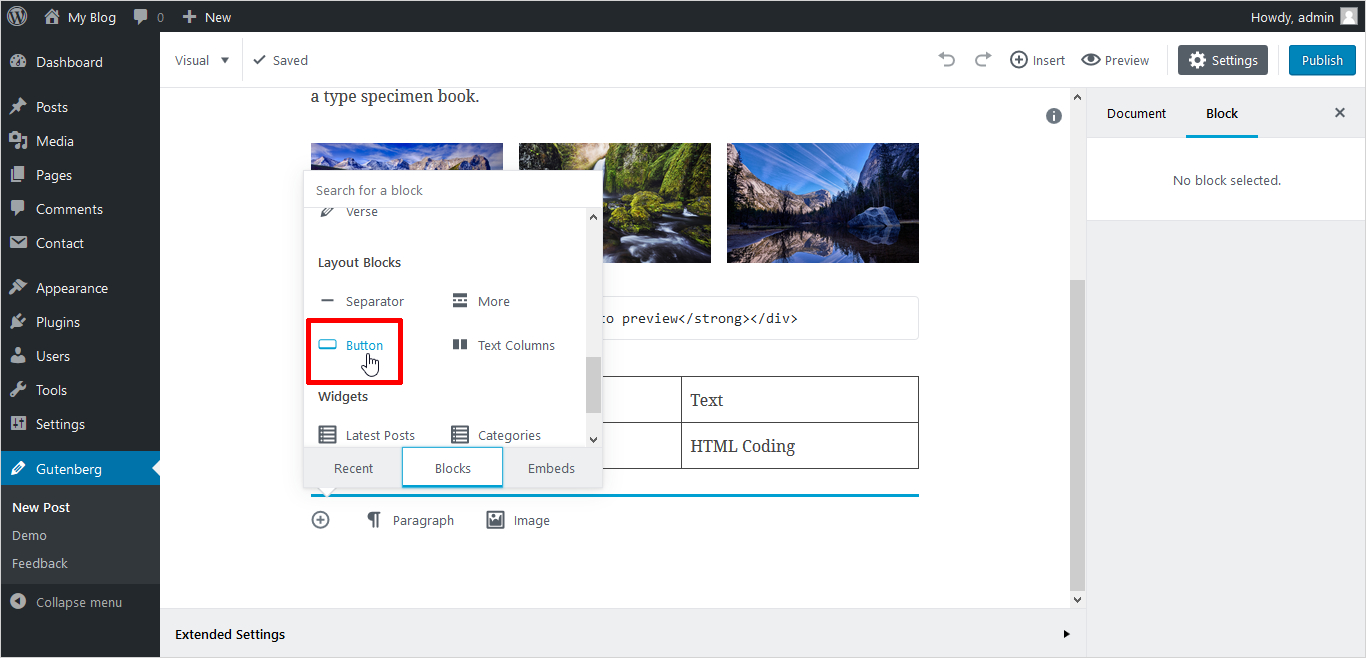A screenshot of a WordPress webpage in editing mode is displayed. The left sidebar, featuring a black background and white text, lists various menu options: Dashboard, Posts, Media, Pages, Comments, Contacts, Appearance, Plugins, Users, Tools, Settings, "Hood and Back" (highlighted in blue), New Post, Demo, Feedback, Collabs, and Mail. 

On the right side, which has a white background, the main content area layout is shown. A clicked option is visible with a search field for blocks and other layout elements such as separator, more, text, and columns. A button, highlighted in blue and outlined in red, is indicated by a hand cursor, while other options remain grey. Below this, the menu displays sections labeled Recent, Blocks (which is highlighted in white), Embeds, and a list that includes Paragraph and Image options.

In the top right corner of the page layout, there is a toolbar with entries labeled Insert, Preview, Settings, and Publish; the Settings button is grey, while the Publish button is blue. Below this, a message reads "No block selected." Illustrative elements include images of mountain landscapes with green fields, rivers, blue skies, and brown rocks interspersed throughout. An extended settings option and a table are located at the bottom left of the screen.